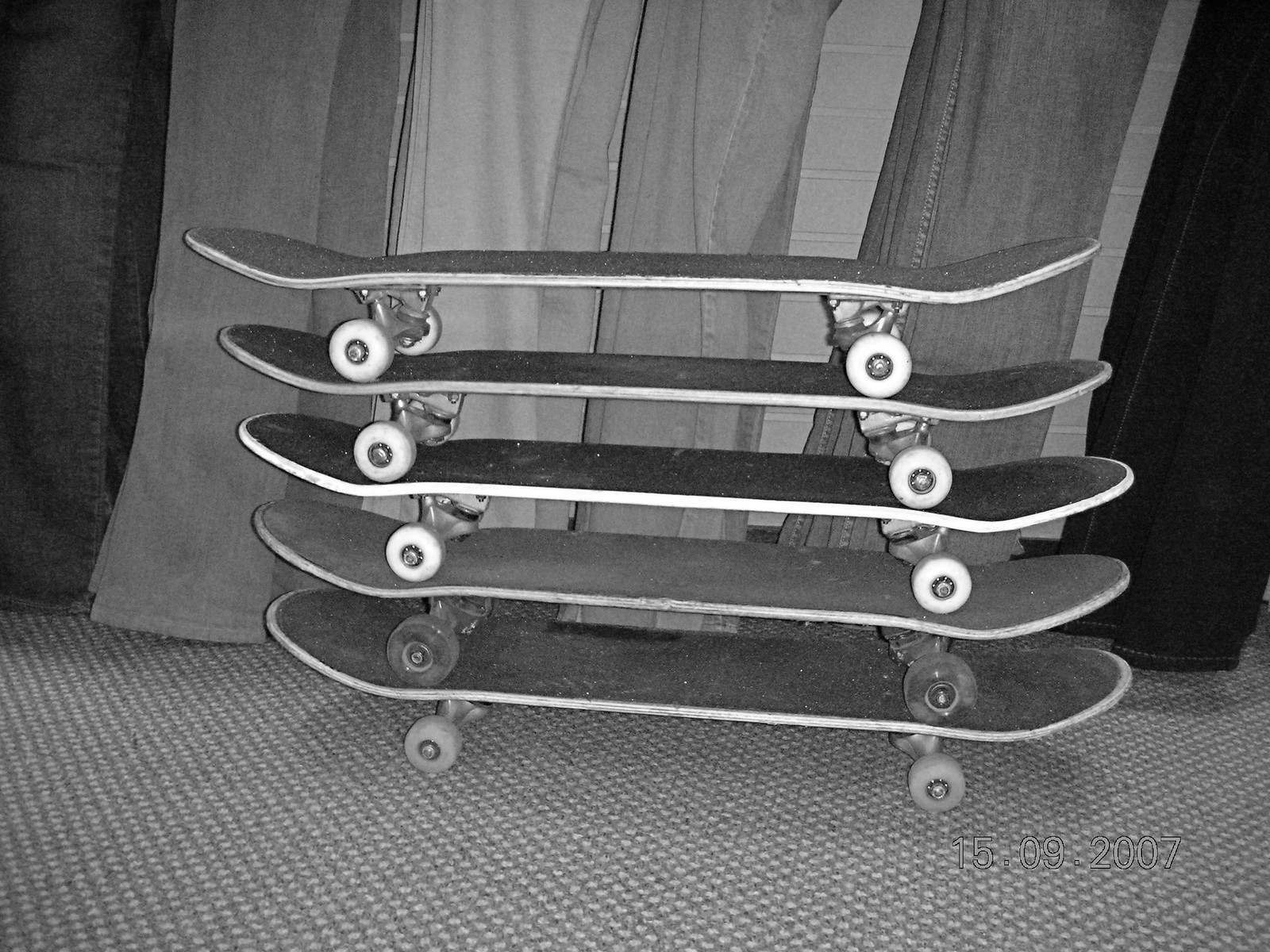This black-and-white photograph, dated 15.09.2007, captures a scene featuring five skateboards stacked neatly on top of each other. The skateboards are arranged so that they rest upright, wheels to board, on what appears to be a gray Berber carpet. The boards themselves feature a rough sandpaper texture, typical of skateboards, with the top three displaying white wheels and the bottom two showcasing wheels in varying shades of gray. Behind the stack of skateboards, a backdrop of jeans—draped in different shades of denim—hangs over a white brick wall, adding a textured contrast to the image's foreground. The minimalist yet detailed composition emphasizes the juxtaposition between the modern urban skateboards and the casual denim elements in the background.